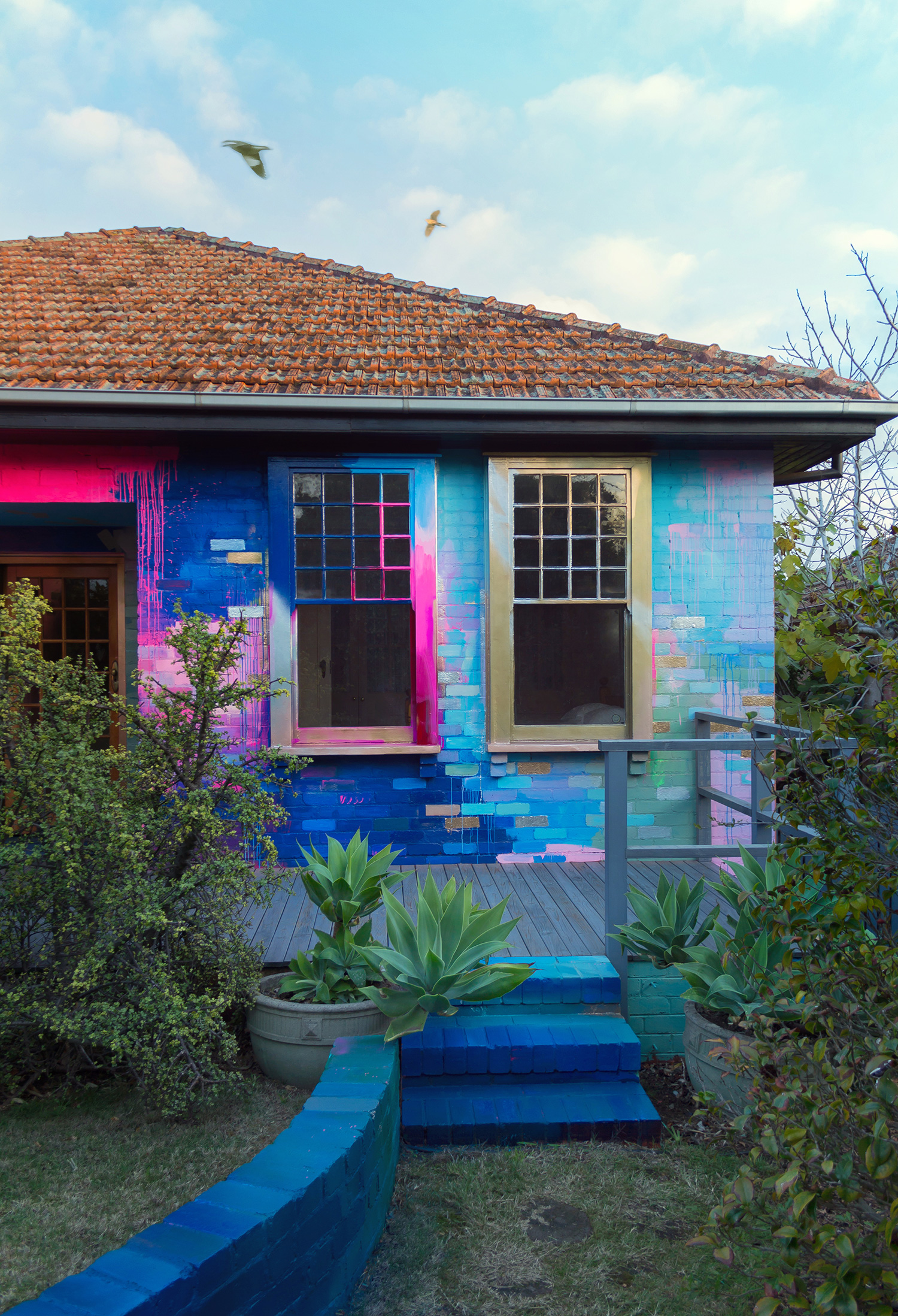This image showcases the vibrant and eclectic exterior of a small ranch-style house. The façade is a colorful mosaic of painted bricks, with shades of light and dark blue, pink, white, and brown, giving it a kaleidoscope effect. The house features an orange clay roof with a triangular design, typical of warm climates. 

The back of the house includes a gray wood deck with a wooden railing, reached by three low brick steps painted in bright blue. One windowsill is adorned with a mix of blue, pink, and gray, while the other sports a yellowish gold hue. Above the door, there are streaks of pink paint adding to the creative chaos.

On the right side of the house, different plants and trees frame the scene, while a small blue-painted brick wall on the left side hosts a gray planter overflowing with green foliage. The yard in front is lush with green grass, and bushes frame the house on both sides. To complete this whimsical outdoor setting, a few birds can be seen flying above, adding a sense of liveliness to the already animated scene.